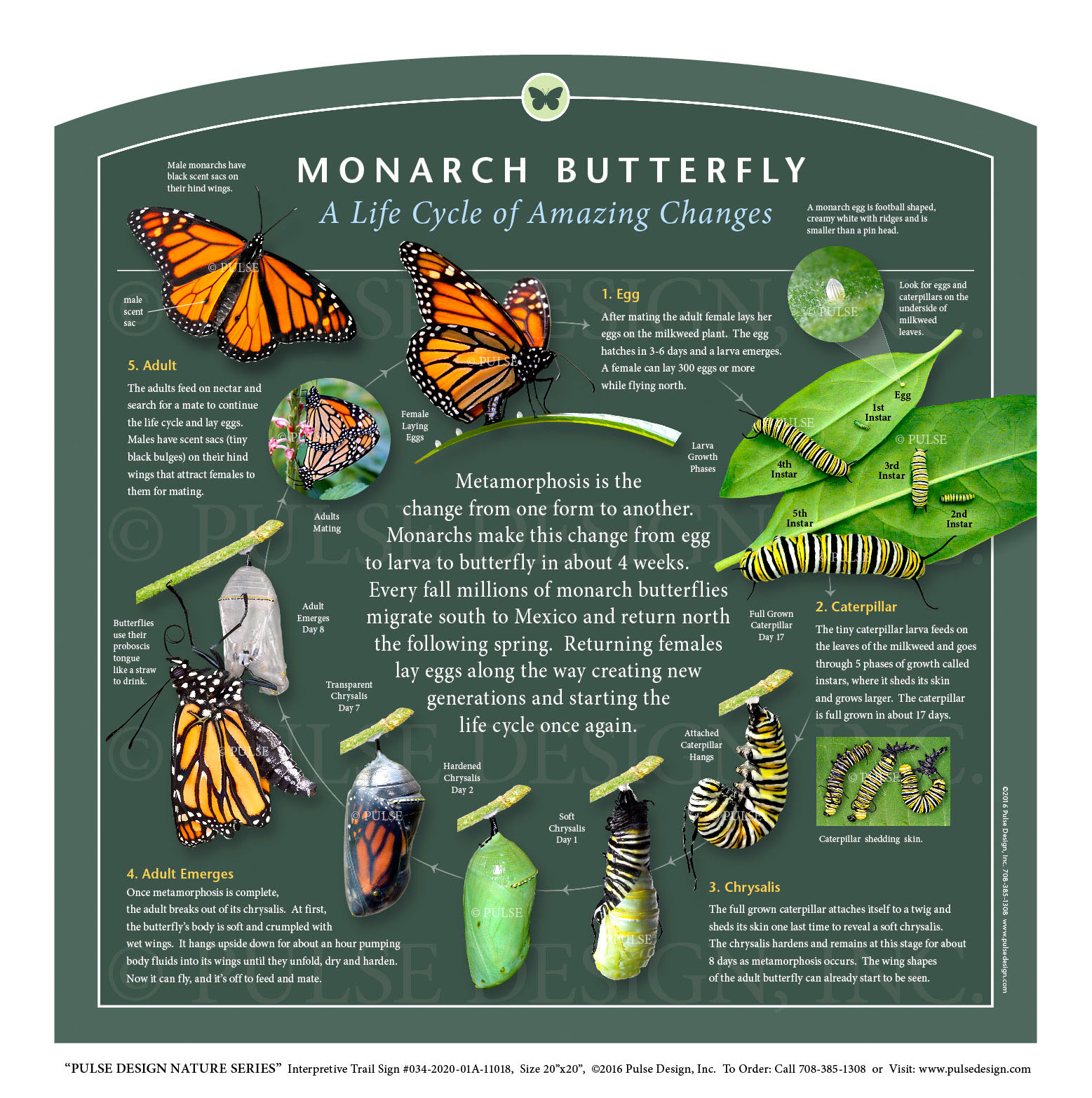A vibrant, dark green poster titled "Monarch Butterfly: A Life Cycle of Amazing Changes" features a comprehensive, clockwise portrayal of the monarch butterfly's life stages. The chart meticulously details the metamorphosis process, explaining the transformation from egg to larva to butterfly, which occurs over approximately four weeks. Central to the poster is a description emphasizing metamorphosis as a fundamental change from one form to another. Surrounding this text are vivid images and descriptions of each stage—egg, caterpillar (or larva), chrysalis, and adult butterfly—accompanied by colorful photographs and illustrations that highlight the vibrant journey of the monarch.

Further details elaborate on the impressive migratory behavior of monarch butterflies: every fall, millions travel southwards to Mexico, returning north in the spring. Throughout this migration, females lay eggs along their route, perpetuating the cycle. The poster beautifully captures the dynamic sequence of the monarch's development, with bright, living colors and detailed illustrations of each life stage, showcasing the species' extraordinary life cycle and seasonal migrations.